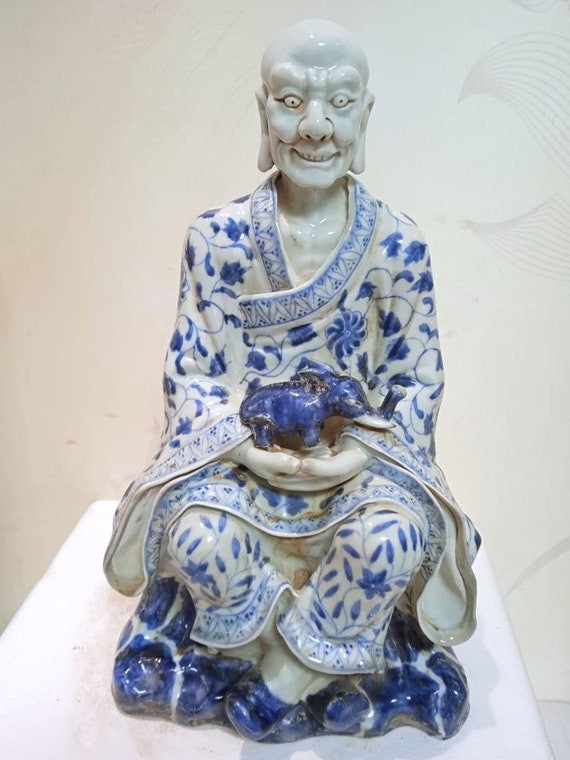The image depicts a ceramic or porcelain statue of a Buddha-like figure with exaggerated and eerie features, sitting on a white platform set against a white painted wall adorned with faint, swirly patterns. The statue has a bald head, long, prominent earlobes, buggish eyes with tiny pupils, deep labial folds around its mouth, and a creepy grin that lends the face a devilish appearance. Unlike traditional depictions of a laughing Buddha, this figure is slender with an elongated head. It is clothed in a long, white robe adorned with blue floral and vining patterns, matching its pants and blue shoes. The statue is seated cross-legged and cradling a small, intricately detailed blue object resembling a baby elephant. This delicate composition is unified by a consistent blue and white color scheme, extending even to the blue-tinted, stool-like base on which the figure perches.